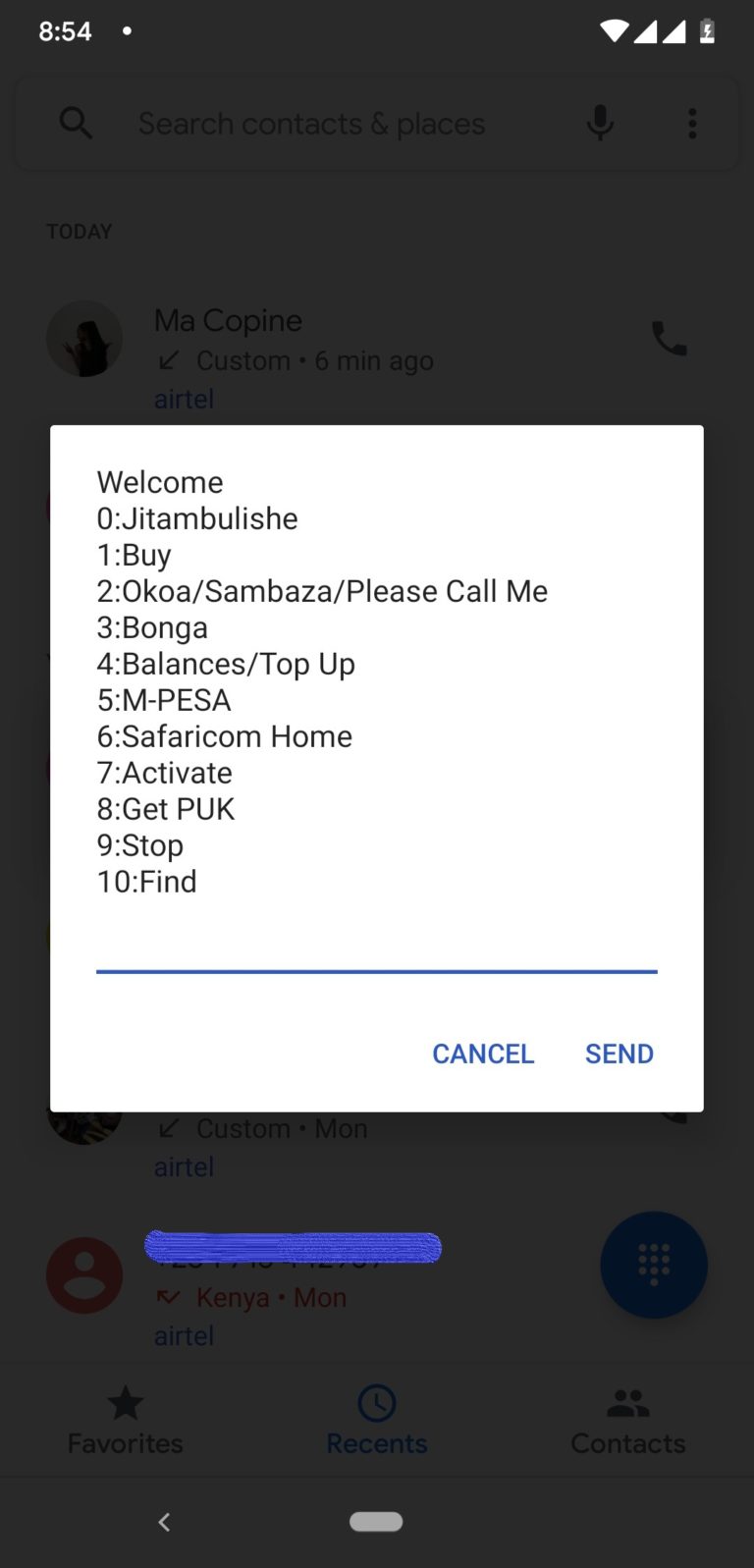A screenshot of a smartphone interface prominently features a white pop-up dialog box that partially obscures the background screen, which includes icons for "Favorites," "Recents," and "Contacts." Below the white box is a bright blue strip displaying the time as 8:54. The dialog box presents a list of options:

1. Welcome
2. 0: Jittaboleeshee
3. 1: Bye
4. 2: Okawisambasa please call me
5. 3: Bonga
6. 4: Balances/Top up
7. 5: MPesaSafaricomHome
8. 7: Activate
9. 8: Get Puke
10. 9: Stop
11. 10: Find

At the bottom of the dialog box is a long light blue line. On the right-hand side, beneath this line, there are two buttons: "Cancel" and "Send."